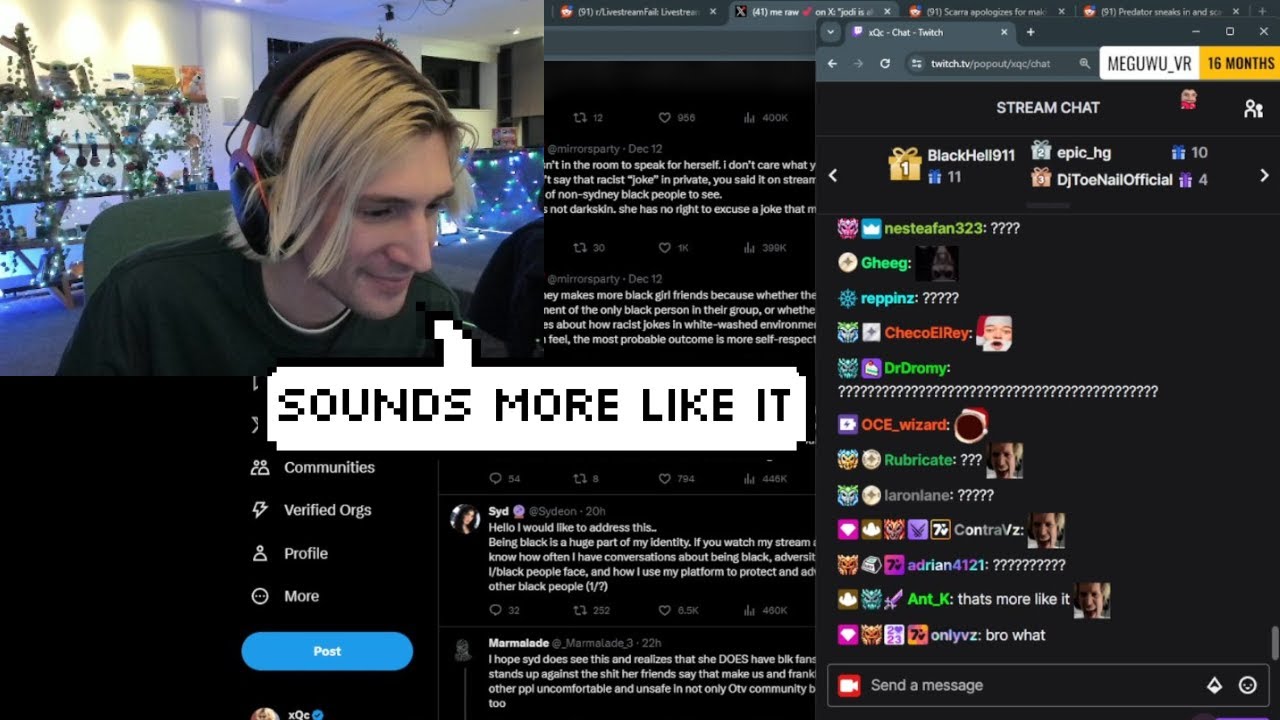This image is a composite screenshot featuring a gaming streamer with blonde, shaggy hair, sporting a pair of headphones and a cheerful smile. The streamer is depicted with a pixelated speech bubble emanating from his mouth, containing the text "Sounds more like it." The overall setting appears to be related to Twitch, as indicated by an open window displaying "Twitch" and "Twitch TV" within an icon.  

Additionally, the screenshot showcases text from the stream chat where the username MEGUWU_VR and "16 months" are visible, surrounded by various messages composed entirely of question marks. Below the chat, there's a snippet that discusses comments possibly attributed to a controversy around racism against black people. This snippet includes text that is too small to read clearly but seems to be a screenshot from the social platform "X," as noted by the visible X icon and terms like "communities," "verified orgs," "profile," "more," and "post." 

The streamer's image is prominently overlaid in the upper left-hand corner of the screenshot, integrating the various elements into what appears to be a complex, layered composite of different platforms and interactions.